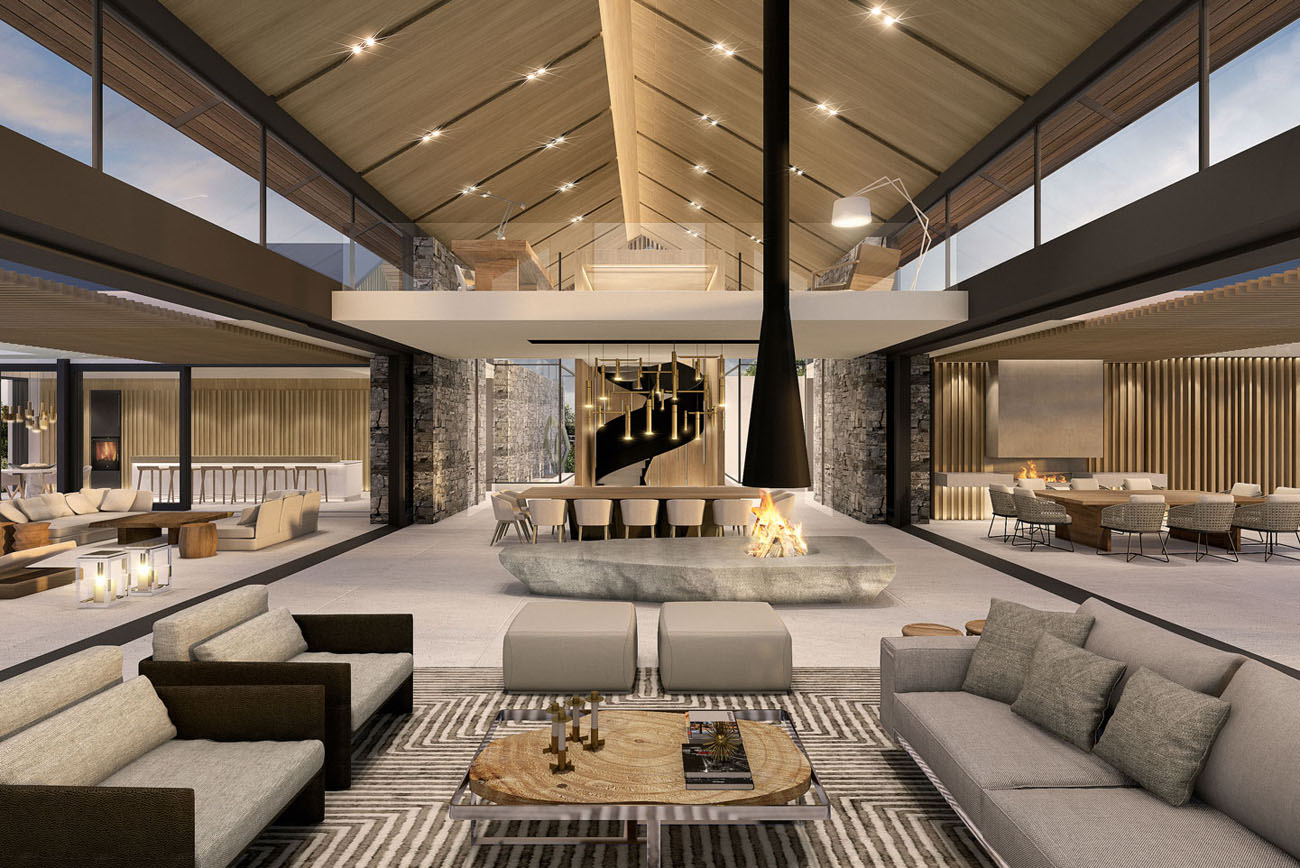This photograph captures the sophisticated atmosphere of an upscale and modern lounge area, likely within a high-end hotel or a lavish modern residence. Dominated by clean lines and minimalistic design, the open space is illuminated by abundant natural light streaming through expansive second-story windows. The ceiling, pointed and triangular, adds a striking architectural feature with built-in LED lights.

Central to the room is a dramatic marble fireplace with a sculptural quality, complete with a black flue extending to the ceiling. Surrounding this focal point are plush gray sofas, accompanied by a distinctive coffee table made from a sliced tree trunk encased in metal and glass, adorned with books and candles for a cozy touch.

To the left, multiple seating areas create an inviting social space with additional couches and tables, while the right side features a substantial dining table encircled by numerous chairs, suggestive of formal gatherings or meetings. The white floor interspersed with two bold black stripes enhances the sleek aesthetic. 

In the background, a spiral staircase ascends to an indoor balcony with glass railings, providing additional seating and tables. This elevated area overlooks the entire lounge, reinforcing the theme of openness and connectivity within the space.